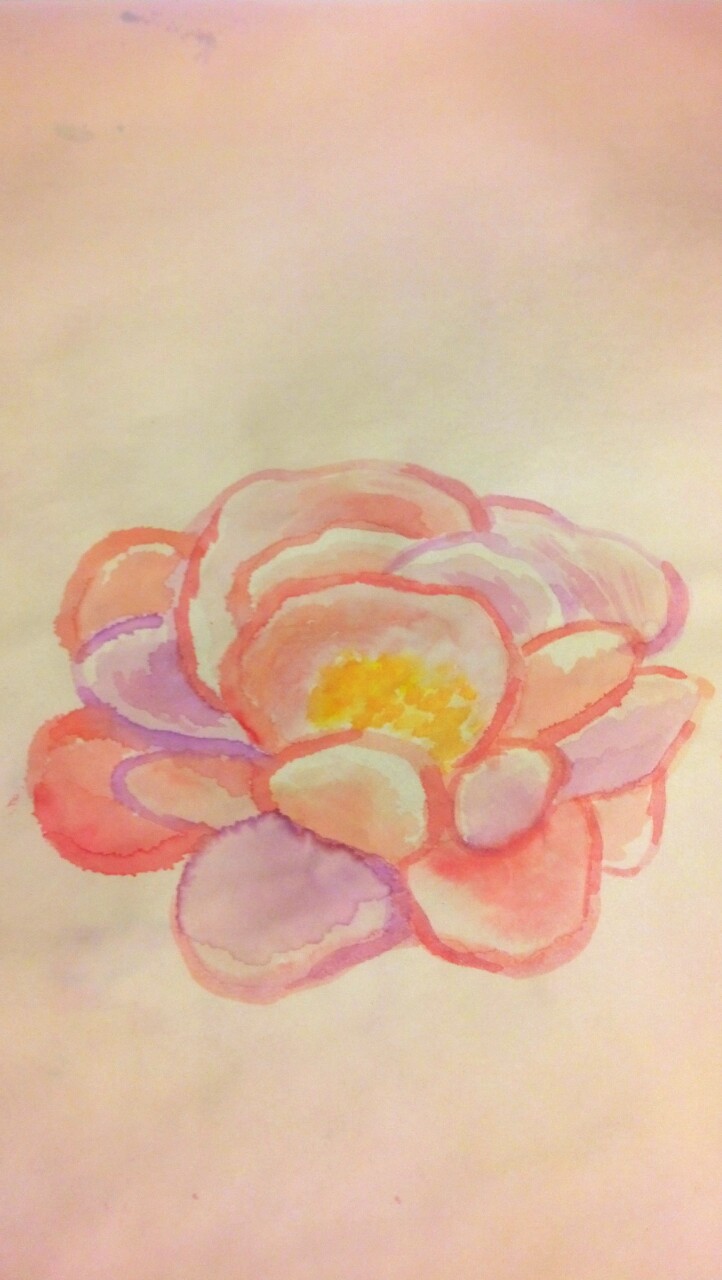A vertically-oriented watercolor or gouache painting showcases a single, exquisite rose at the center. The background features a soft wash of pastel hues, seamlessly blending light orange, pink, and green into a cohesive, serene backdrop. The rose itself is delicately outlined in shades of pink and red, with its petals infused in harmonious tones of pinks, reds, and purples. The heart of the flower, perhaps symbolizing its pistil, transitions from a gentle light yellow to a rich, dark yellow. The absence of leaves or a stem focuses all attention on the intricate beauty and vibrant colors of the rose, making it the undeniable focal point of this captivating artwork.